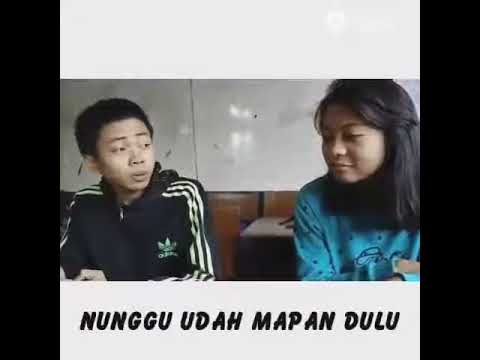The image portrays two young individuals engaged in conversation. The male on the left, who appears to be of Asian descent, has short black hair and is wearing a dark blue or black Adidas sweater with white stripes on the arms. His mouth is slightly open as if he’s speaking to the female. The female, also appearing to be Asian, has shoulder-length black hair, a blue shirt, and seems to be looking towards the male with her eyes partially closed. They both appear to be in their late teens, suggesting an age range of 15-20 years.

The background includes what seems to be a whiteboard with smudges and a brown wooden trim below, indicating a casual setting that may be an educational or informal space. The photograph is presented in a landscape orientation and inset into a white background, which is further bordered by black strips on both sides. At the bottom of the image, there is a section with black text on a white background that reads “N-U-N-G-G-U-U-D-A-H-M-A-P-A-N-D-U-L-U,” suggesting the inclusion of a foreign phrase or word.